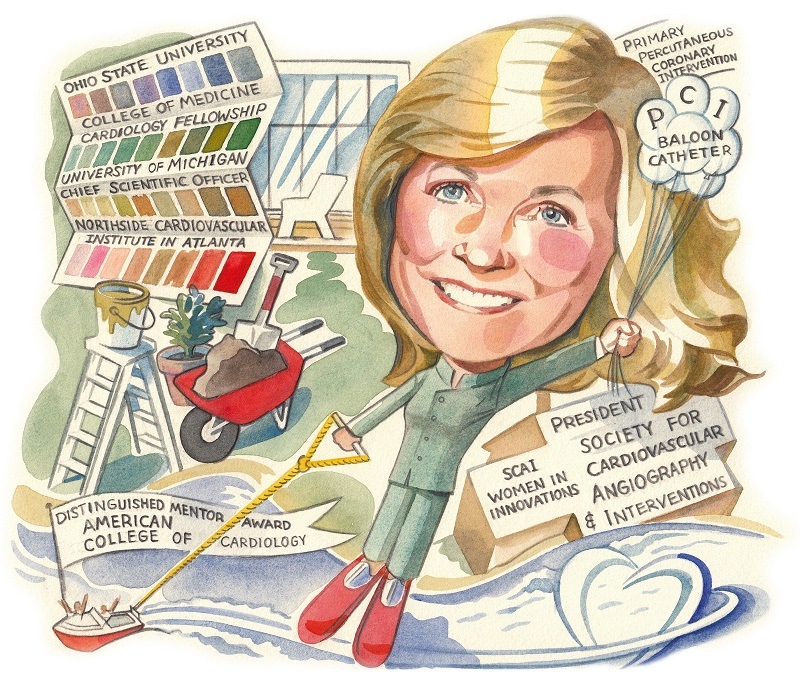This vibrant caricature showcases a cheerful woman with an oversized head of blonde hair, blue eyes, and rosy cheeks. She is dressed in a button-down, long-sleeve green shirt with a Chinese collar, matching green pants, and unusually large red shoes. The woman is smiling broadly as she clutches a bunch of balloons labeled "PCI balloon catheter" in her left hand. In her right hand, she holds a cord, similar to a water ski rope, tethered to a boat. This boat displays a banner proclaiming "Distinguished Mentor Award, American College of Cardiology."

Directly to her side, multiple items cluster together: a wheelbarrow full of dirt with a shovel, a potted plant, a white ladder with olive green paint spilling over its sides, and a fan of paper containing numerous color swatches and text. The text on the paper reads "Ohio State University College of Medicine, Cardiology Fellowship, University of Michigan, Chief Scientific Officer, Northside Cardiovascular Institute in Atlanta."

Set behind the fanned paper is a window framed with a white chair. Above her, the words "Primary Percutaneous Coronary Intervention" are prominently displayed. To her left, a top-down view of a house bears the inscriptions "SCAI Women in Innovations" and "President, Society for Cardiovascular Angiography and Interventions."

This dynamic and detailed scene unfolds against a backdrop of blue waves, on which the caricatured woman appears to be water skiing, encapsulating a lively fusion of her professional accolades and whimsical, comic illustration style.